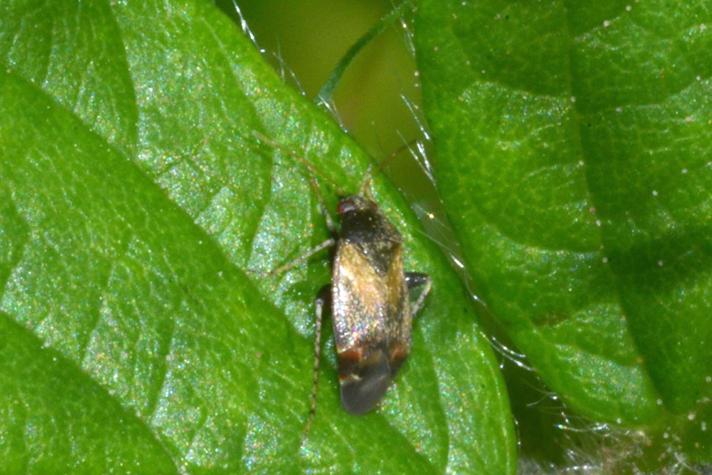This horizontally aligned color photograph, likely taken outdoors during daylight, captures a detailed, close-up view of a black and gold beetle perched on one of two green leaves from the same plant. The photograph showcases these leaves, rich in a royal green hue, displaying fine, silvery hairs along their lobes and veins, with sunlight reflecting off these delicate fibers.

The beetle, prominently perched on the left leaf, has a predominantly black body adorned with a gold back that might be its folded wings or a shiny shell. The beetle features a small black head, large black eyes, and six legs; its back legs are long and bent, middle legs shorter, and front legs long and skinny with possible white and black striping. The head area also sports a pointed feature and possible antlers. The intricate details of the beetle's body include a silver V-shaped mark, colorful speckles, and a transition from gold to brown and then black towards the tail end.

Enhancing the image’s green background, hints of orange can be seen peeking through the leaves' gaps, emphasizing the lush and vibrant environment. This photograph, with its scientific accuracy and clarity, could easily be featured in a nature magazine.